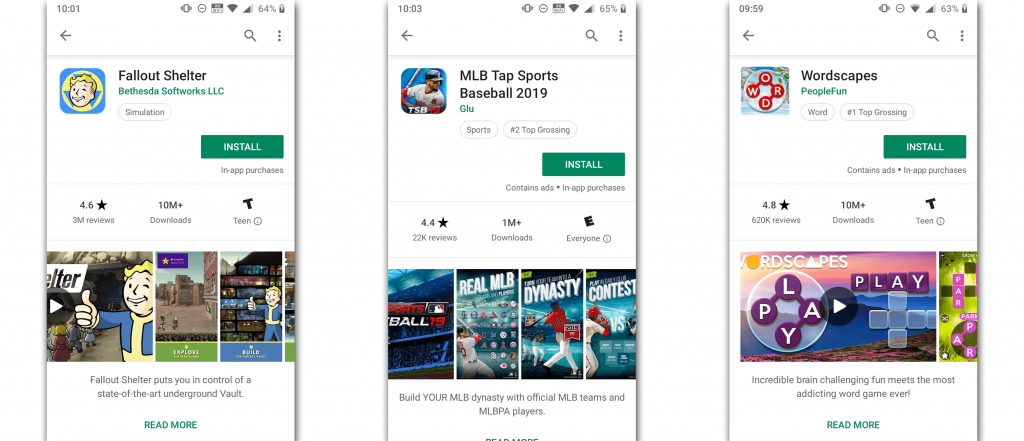The image is divided into three distinct panels, each representing a different mobile phone screenshot against a white background. Here is a detailed breakdown of each panel:

**Left Panel:**
- **Header:** The time displayed at the top is 10:10 AM, accompanied by typical phone status icons such as a vibrating phone icon, cell signal strength, Wi-Fi signal, and battery level at 64%.
- **Navigation & Information:** Below the status icons, there's a back arrow, a search icon represented by a magnifying glass, and three vertical dots indicating a menu.
- **App Details:** The app shown is "Fallout Shelter" by Bethesda Softworks LLC. It falls under the 'Simulation' category.
- **Install Button:** A prominent green button labeled "Install" in white text, indicating the availability of in-app purchases.
- **Ratings & Downloads:** The app is rated 4.6 stars based on 3 million reviews, and it has over 10 million downloads. The content rating is 'T for Teen.'
- **Game Description:** A brief description beneath graphics showcasing various scenes from the game reads, "Fallout Shelter puts you in control of a state-of-the-art underground vault." There is also an option to "Read More."

**Middle Panel:**
- **Header:** The time is 10:03 AM with similar phone status icons.
- **Navigation & Information:** This panel also includes a back arrow, a search icon, and three vertical dots.
- **App Details:** The featured app is "MLB Tap Sports Baseball 2019" by GLU in the 'Sports' category, marked as number two in the top charts.
- **Install Button:** A green install button indicating in-app purchases.
- **Ratings & Downloads:** The app has a 4.4-star rating from 22,000 reviews and over 1 million downloads. It is rated 'E for Everyone.'
- **Game Description:** The description highlights, "Build your MLB dynasty with official MLB teams and MLBPA players," with accompanying game graphics.

**Right Panel:**
- **Header:** The time shown is 9:59 AM, with the same set of status icons.
- **Navigation & Information:** Includes a back arrow, a search icon, and three vertical dots.
- **App Details:** The app displayed is "Wordscapes" by PeopleFun, labeled as 'Word,' falling under the 'Number one top charts' category.
- **Install Button:** A green install button, similar to the other panels.
- **Description & Graphics:** There are graphics related to gameplay with an option to "Read More."

Overall, each panel meticulously presents key details of different apps, including app names, developers, genres, top chart rankings, install buttons, ratings, download numbers, and descriptions, complemented by visual elements and standard mobile interface icons.